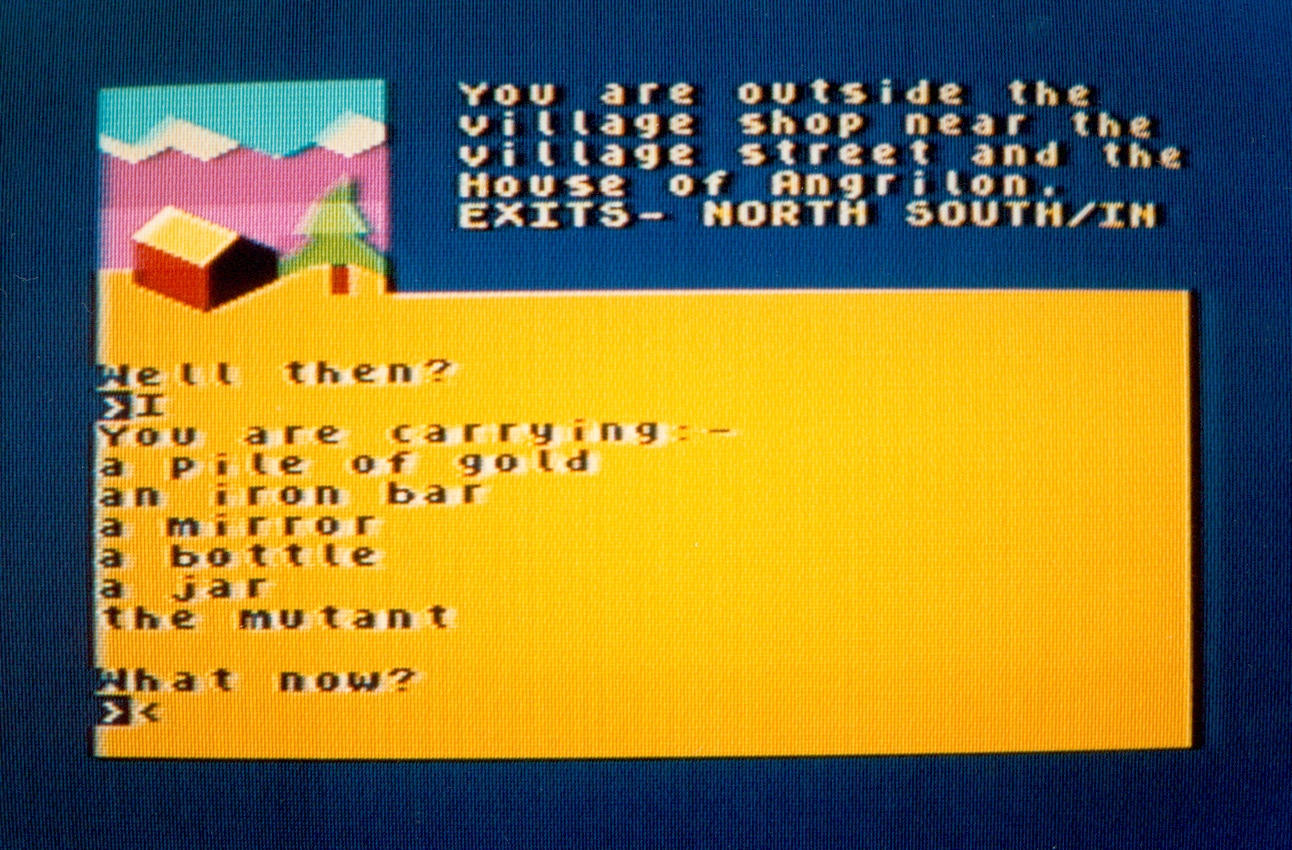A screenshot showcases a nostalgic, pixelated, choose-your-own-adventure game with a vintage aesthetic. The background is a deep blue, while a prominent orange-yellow window occupies the lower half of the screen. In the upper left corner of the window, a charming pixel art scene features a green tree beside an orange-hued house under a blue sky with a pink section.

Adjacent to this image, pixel text reads: "You are outside the village shop, near the village street and the house of Angrilon." Below, in capital letters, "EXITS: NORTH, SOUTH, IN" provides movement options. The orange section beneath the scene displays black text: "Well then," followed by "I," and a list of carried items: "a pile of gold, an iron bar, a mirror, a bottle, a jar, and the mutant." The prompt "What now?" with angle brackets invites the player to choose their next action. The entire composition evokes a sense of adventure and retro gaming charm.